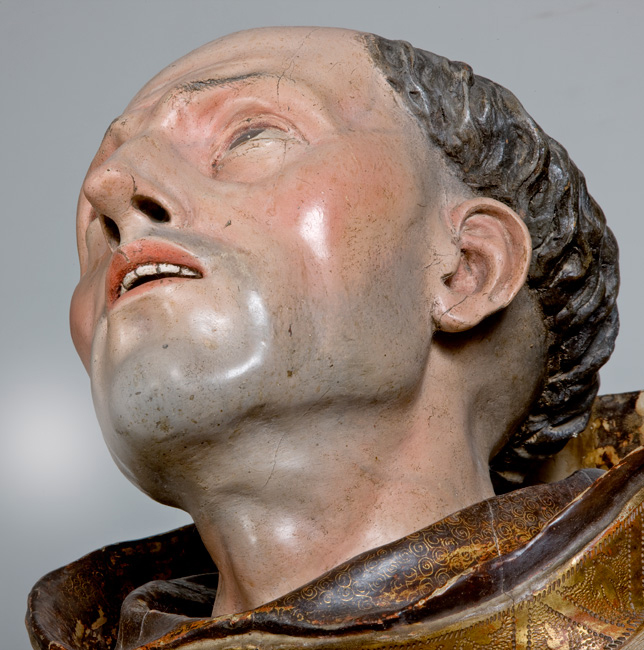The square photograph, measuring approximately five inches by five inches, captures an intricately detailed bust of a monk-like figure against a plain gray background. The statue portrays a Caucasian man with light, pinkish skin and a distinctive five o'clock shadow. His large forehead and pointed nose are directed towards the upper left corner, giving him an expression that seems a mix of awe and resignation.

His hair is grayish-brown, curling under at the sides and temples while bald on top, and is slightly shaved above and behind the ears. Gray eyes look upward, contributing to his intense expression. The lips are a deep pinkish-red, slightly open to reveal the upper row of white teeth, and the skin tone takes on a pinkish-gray hue near the chin where he likely shaves.

The figure is cloaked in a rich brown cowl adorned with intricate gold engravings, adding a touch of elegance and age to his appearance. The vestment appears heavy and textured, reminiscent of medieval garments. The overall aesthetic suggests that the bust is a painted wooden sculpture, capturing the serene yet solemn essence of a monk from the 1500s.